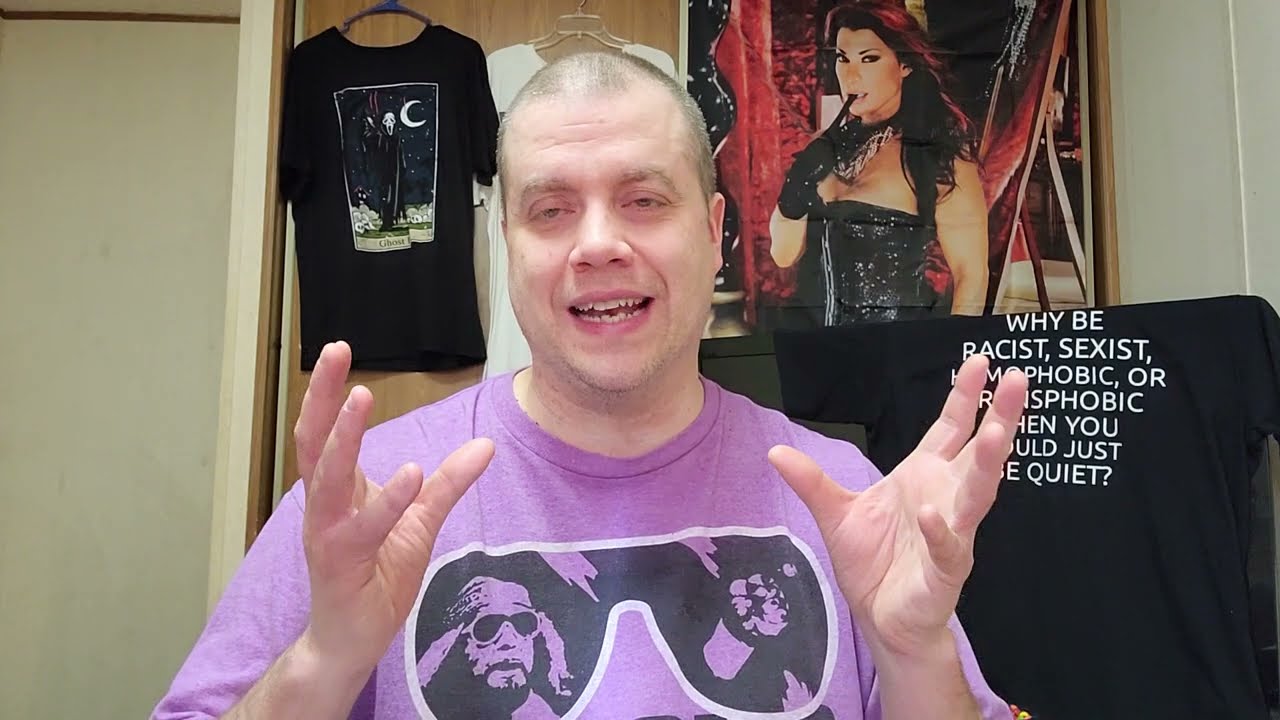The image captures a middle-aged, balding Caucasian man with short, graying hair and heavy-lidded eyes, who is speaking animatedly to the camera with his hands raised. He is wearing a lavender, short-sleeved shirt that features a graphical design of a pair of sunglasses. Inside one of the sunglasses’ lenses, there appears to be an image reminiscent of a wrestler, possibly Macho Man Randy Savage. Behind the man, in what appears to be a dorm or apartment room, a few items of interest are visible on the wall. Directly behind him hangs a poster of a woman who resembles a movie star, dressed in a black dress and black gloves, and possibly striking a dramatic pose. To the right of this poster is a black t-shirt draped over a wooden surface, and below this is another black t-shirt with white lettering that reads, "Why be racist, sexist, homophobic, or transphobic when you can just be quiet?" The man’s expressive demeanor and the eclectic decor give the room a distinctly personal and idiosyncratic atmosphere.